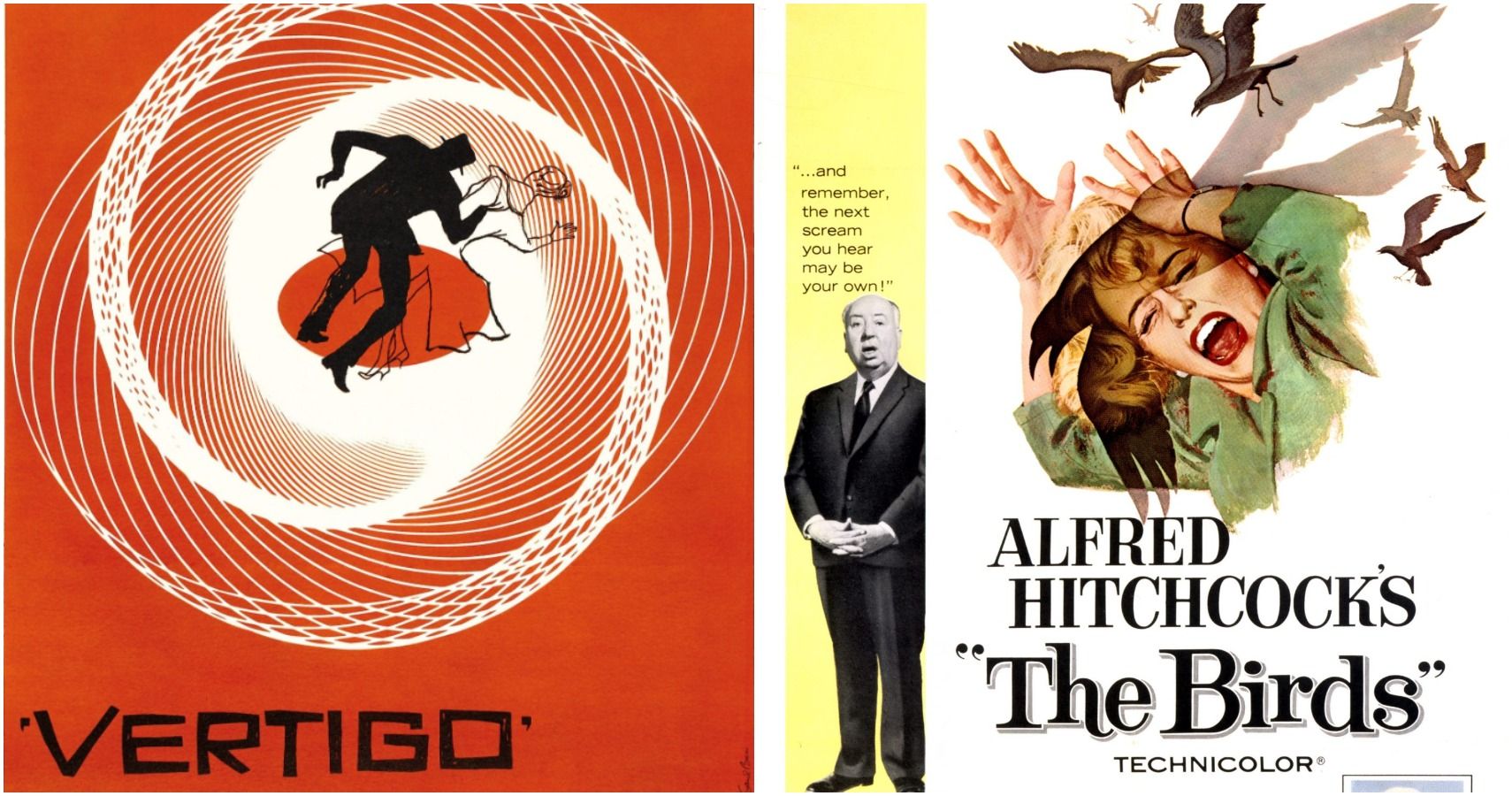Here we have a horizontally rectangular piece featuring two square, vintage movie posters of Alfred Hitchcock's iconic films. The overall image is divided by a thin white line with no other border. The left poster, set against a bold reddish-orange background, is for the movie "Vertigo." It depicts an intricate white spiral with two central silhouettes: a delicately rendered white figure of a woman, leaning back in an almost dance-like pose, tangled with a fully blackened silhouette of a man. At the bottom, the title "Vertigo" is displayed in large, menacing uppercase letters, with a small, vertical strip featuring a black-and-white photograph of Alfred Hitchcock in his classic dark suit, clasped hands, and slightly open mouth, above the iconic quote, "And remember, the next scream you hear may be your own."

The right poster primarily features a stark white background with a yellow strip on the far left. It advertises "Alfred Hitchcock's The Birds," showcasing an artistic, colored interpretation of a woman in a green overcoat, her mouth open in a scream, fending off a flurry of attacking birds. The birds are depicted with sharp beaks and menacing wings, surrounding the terrified protagonist and capturing the essence of chaos and fear. Below her, "Alfred Hitchcock's The Birds" is written in bold black letters, with "Technicolor" noted in small caps beneath.